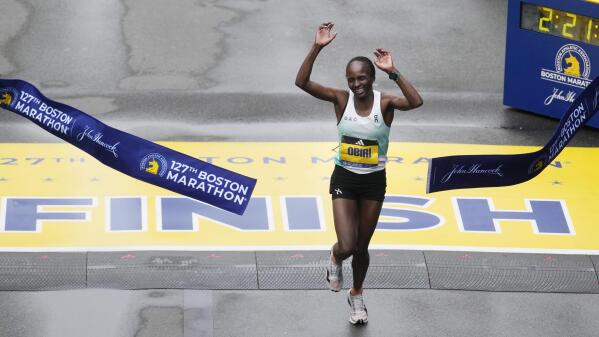This vibrant color photograph captures the triumphant moment of a dark-skinned female runner, Obidi, crossing the finish line of the 127th Boston Marathon. She bursts through a blue banner emblazoned with "127th Boston Marathon" in white letters, her hands raised high and a broad smile illuminating her face. Behind her, the ground features a large, yellow painted strip with "Finish" written in blue letters, accented with a white outline at the bottom. Obidi is dressed in a white tank top with green accents, black spandex shorts, and light-colored sneakers with darker stripes. She sports a watch on her right wrist. The street pavement appears slightly damp, perhaps from recent rain. In the upper right corner of the image, a digital timer displays “2:21.” The background shows an empty, rain-kissed street, focusing all attention on the marathoning champion's moment of victory.